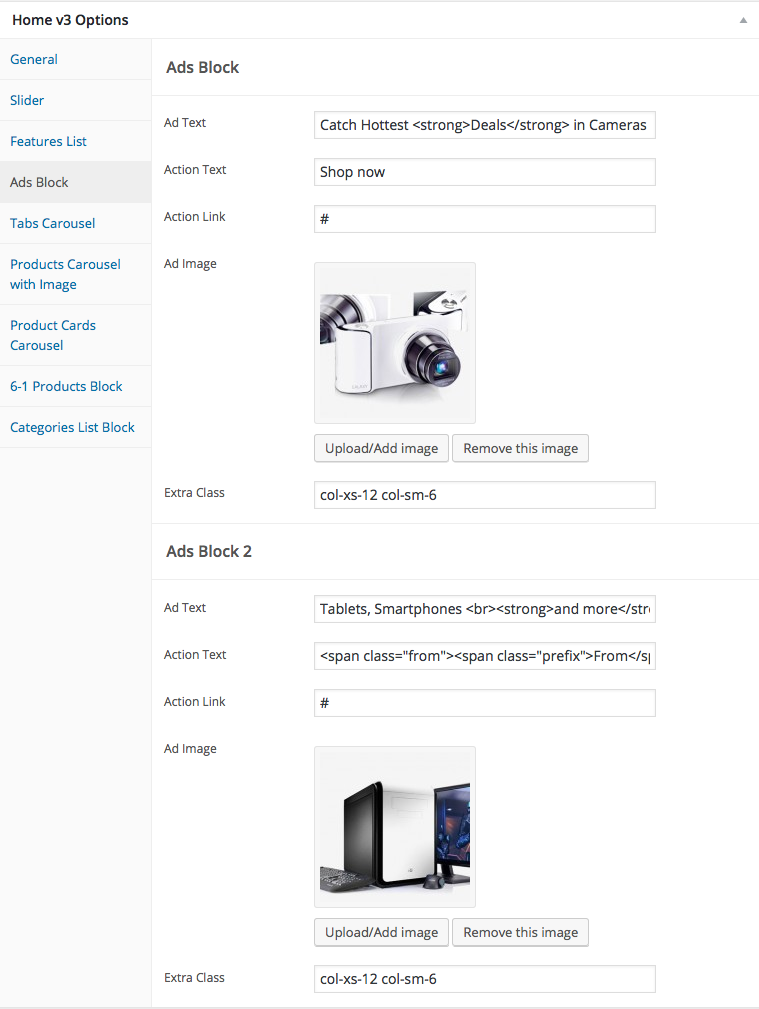**Detailed Caption:**

The image is a screenshot from a mobile application menu, featuring a predominantly white background. At the very top, there is a white bar with the text "Home v3 Options" displayed in a clear black font. Below this bar, a vertical list in blue font is presented, containing several menu options: "General," "Slider," "Features List," "Ads Block" (highlighted and selected), "Tab Carousel," "Product Carousel with Image," "Product Card Carousel," "Six and One Products Block," and "Categories List Block."

The selected menu option, "Ads Block," opens a new section. This section also features a white background and is titled "Ads Block" at the top. Below this heading, two ad configuration blocks are displayed. 

The first ad block includes:
- **Ad Text:** "Catch hottest <strong>deals</strong> in cameras"
- **Action Text:** "Shop Now"
- **Action Link:** Indicated by a placeholder "hashtag"
- **Ad Image:** Featuring a digital camera
- **Options to:** "Upload Ad Image" or "Remove This Image"
- **Extra Class:** With the values "col-xs-12" and "col-sm-6"

The second ad block includes:
- **Ad Text:** "Tablets, smartphones, <strong>and more</strong>"
- **Action Text:** "<span class='prefix'>From</span>"
- **Action Link:** Indicated by a placeholder "hashtag"

Each ad block component is designed to allow customization of the displayed text, action prompts, links, and images, as well as adjusting layout classes for responsive design.